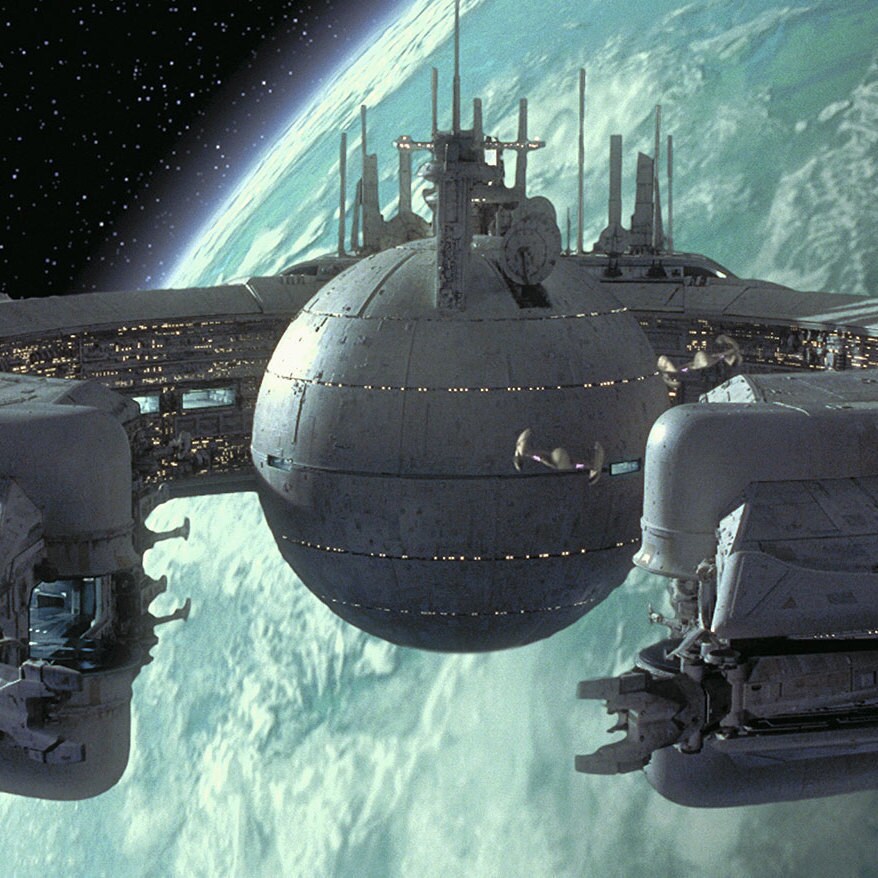In this detailed image, a futuristic space scene is depicted with Earth in the background. The planet, rendered in shades of blue, green, and white, takes up most of this large, borderless square picture. The curvature of Earth can be seen as it cuts across the center of the composition, creating a colorful backdrop of landmasses and atmospheric haze, with a white, translucent smog near the upper regions.

Dominating the foreground is an intricate, spherical space station, reminiscent of spacecraft from Star Wars. This station is primarily gray, accentuated with horizontal lines and numerous small lights, giving it a technological and advanced appearance. The structure includes a central gray sphere surrounded by a circular casing dotted with more illuminated features. The overall design suggests it could be a modular or segmented structure with latches and connecting points.

Additionally, a smaller spacecraft, matching the style of typical sci-fi vehicles, can be seen approaching or docking with the station. This smaller ship is also gray and features tiny lights, contributing to the busy space traffic surrounding the primary structure. 

The upper left corner of the image is a stark contract with its deep blackness, punctuated by numerous tiny white dots representing distant stars, enhancing the feeling of being far from Earth. This space scene evokes a sense of advanced exploration and technology, likely set in a far-off future or a classic science fiction universe.